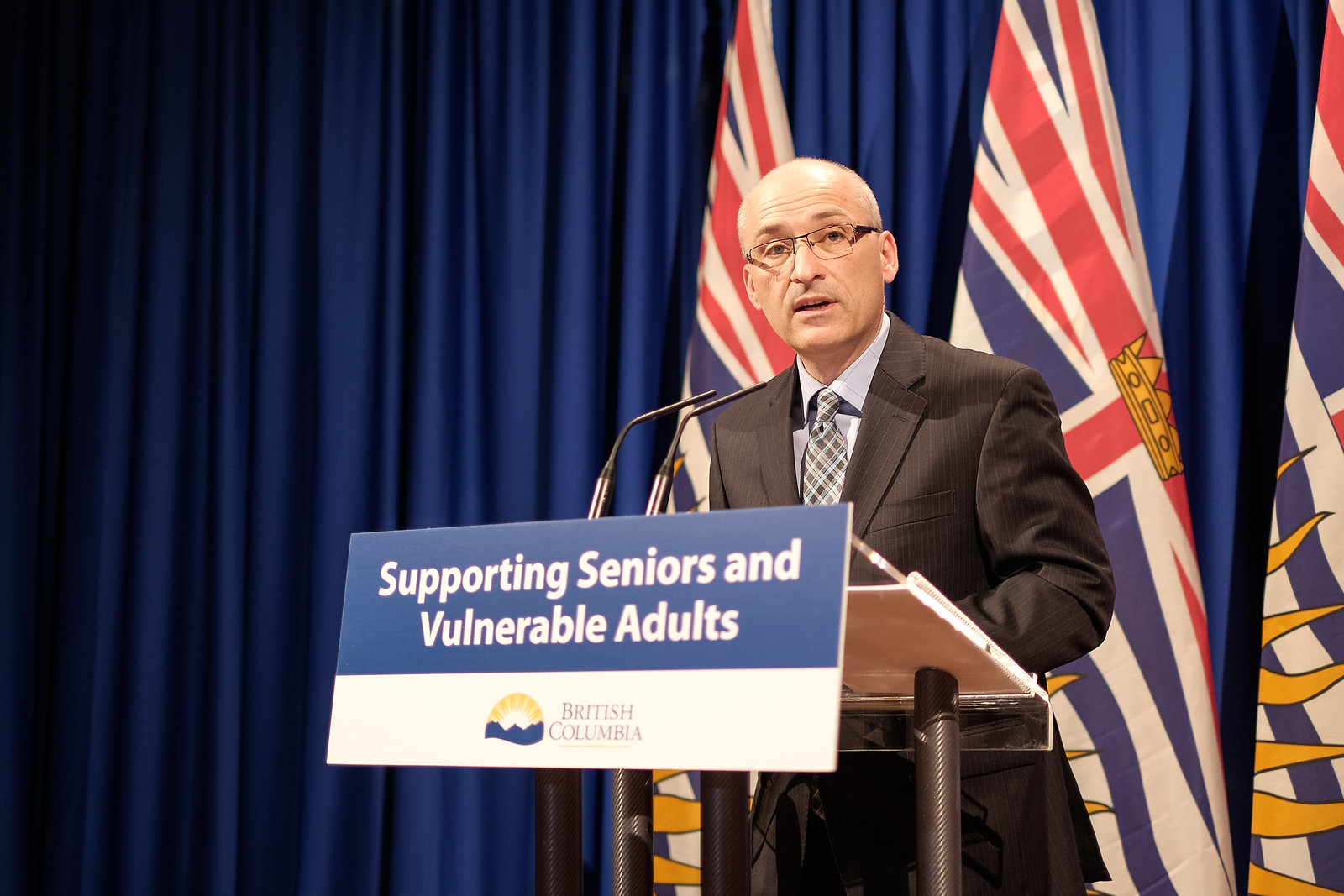The image features a bald Caucasian man standing at a podium giving a speech. He wears a dark grey or black suit, a light blue shirt, and a plaid blue and brown tie, and has glasses on. The podium, which appears to be made of glass or hard plastic with brown pillars, has a prominent sign that reads "Supporting Seniors and Vulnerable Adults" in white letters on a blue background. Below this, a white section of the sign features the text "British Columbia" and a logo depicting a sunset and blue mountains. Behind the man are three flags, likely British Columbian, and a large blue curtain serves as the backdrop. There are two microphones attached to the podium, suggesting that he is in the middle of delivering his speech.